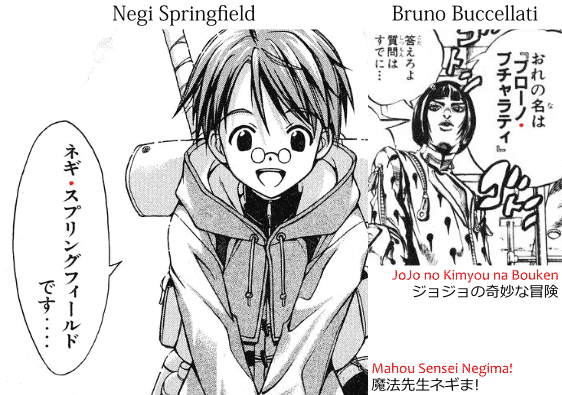The image is an intricate black and white anime illustration marked by certain vivid red text elements. At the center is a boy named Negi Springfield, identifiable by his spiky hair partially covering his face and his small, round reading glasses perched on his nose. He appears curious and surprised, with his mouth agape and eyes looking downward. His hoodie with drawstrings hanging down adds to his youthful appearance. To his left, a speech bubble containing kanji characters emphasizes the Japanese setting.

To the right, a more serious figure, Bruno Bucciarati, is dressed in a coat, with straight hair framing his face and extending down below his chin. Speech bubbles with vertical Japanese kanji surround him, adding depth to the dialogue being depicted.

In the lower portion of the image, two notable texts are written in red. Directly beneath the illustration is the phrase "Jojo no Kimoi na Bokken," followed by horizontal Japanese characters. At the bottom right of the image, the text "Mahou Sensei Negima!" is prominently displayed, also accompanied by Japanese letters.

The overall background is white, providing a stark contrast to the grey, detailed anime characters, which are distinctively drawn. The stylistic elements and the structured placement of text emphasize the intricate and narrative-driven style typical of anime art.